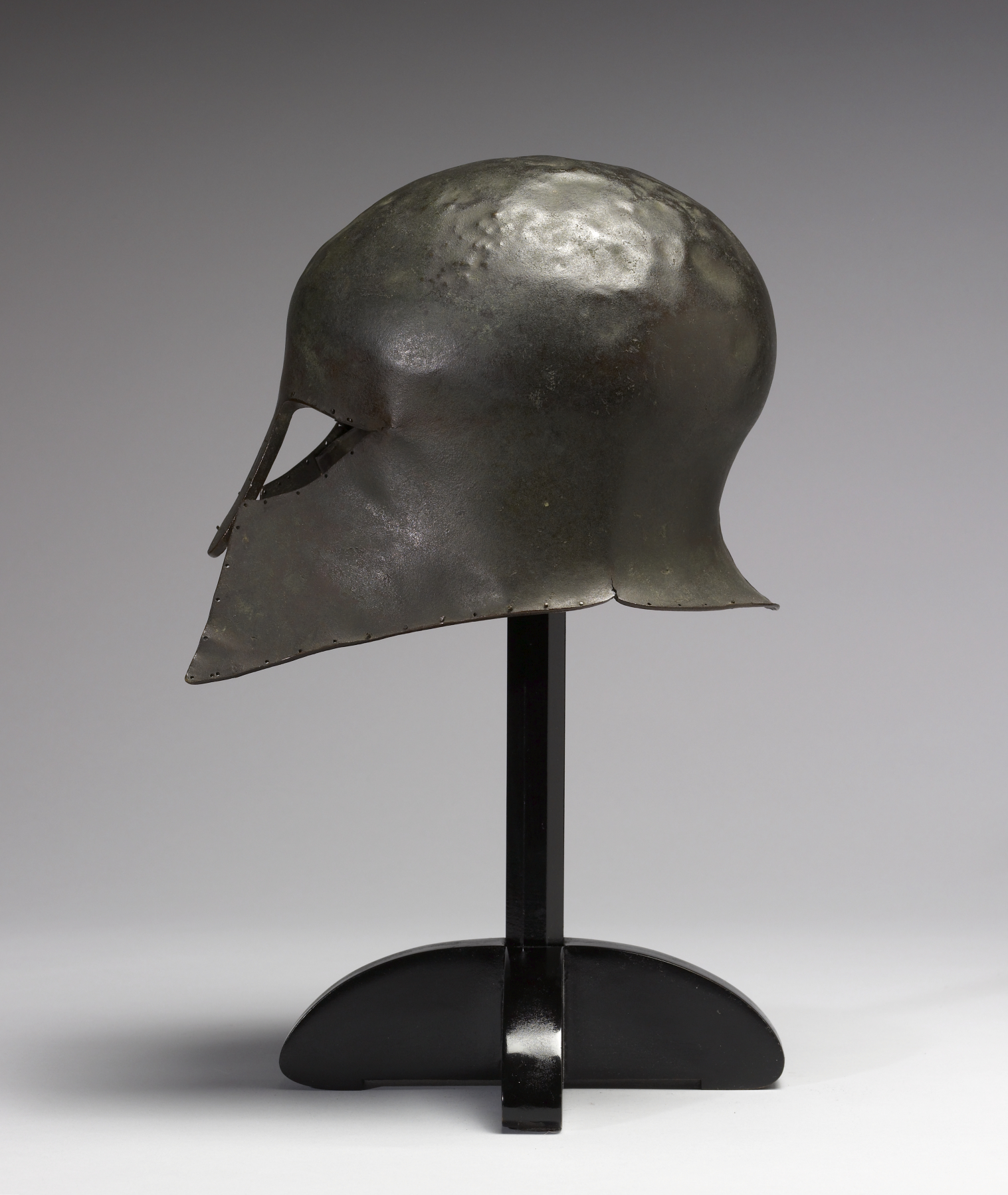This photograph captures an antique, silver metal helmet, possibly Roman or knight's armor, displayed on a wooden black stand with four legs. The helmet, with noticeable hammer marks, exhibits a simplistic design featuring two eye slits and a nose guard flap. It is positioned on a light grey table against a gray and white background, creating a stark contrast that draws attention solely to the helmet and its display. The side profile of the helmet is shown, highlighting its age and craftsmanship. The overall aesthetic, including the gradual gray tones in the background, suggests it could be an exhibit in a museum.